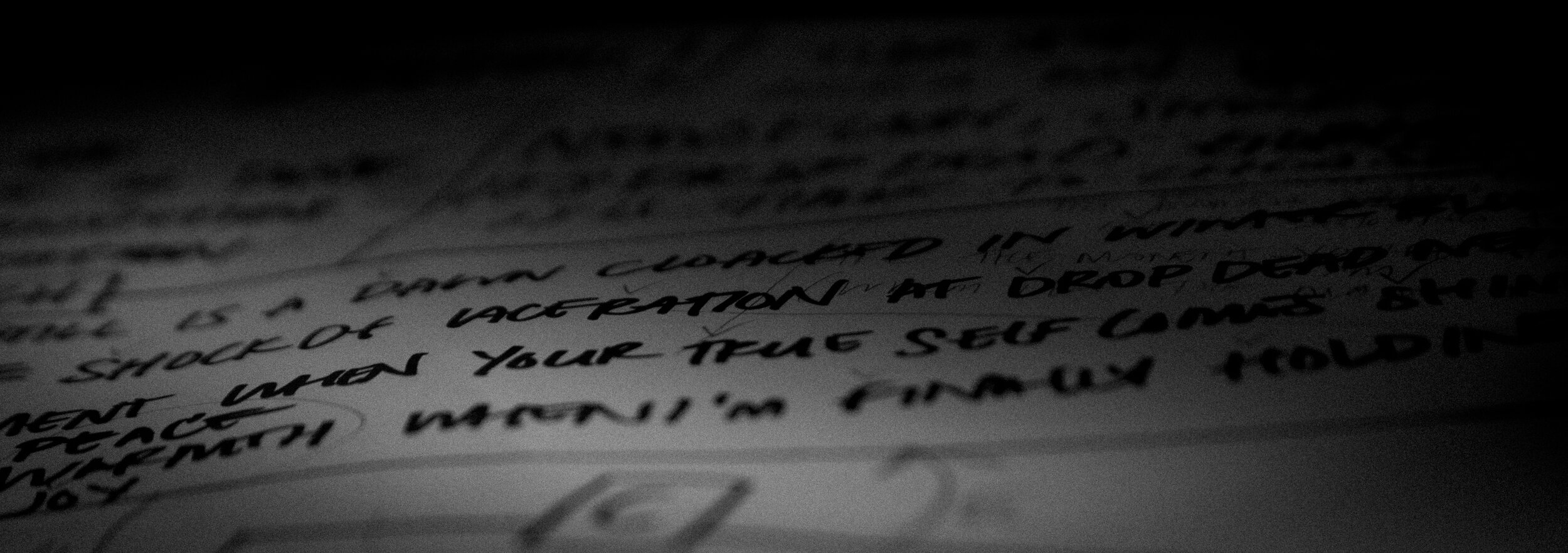This is a horizontally aligned rectangular image that is wider than it is tall. Predominantly black and white, the image is characterized by a dark, almost solid black vignette that envelops the top and stretches down the right side. The focal point is a sheet of lined notebook paper positioned at an angle with approximately ten rows of text written in black marker. Due to the dark vignette and blur effects applied to the image, much of the text is illegible. However, certain phrases can be discerned, such as "is a dawn," "when your true self," and "when I'm finally old." The paper is partially cut off on both the left and right sides, further limiting the visible text to the central portion. The overall tone of the image is deeply shadowed, emphasizing a sense of mystery and obscurity.